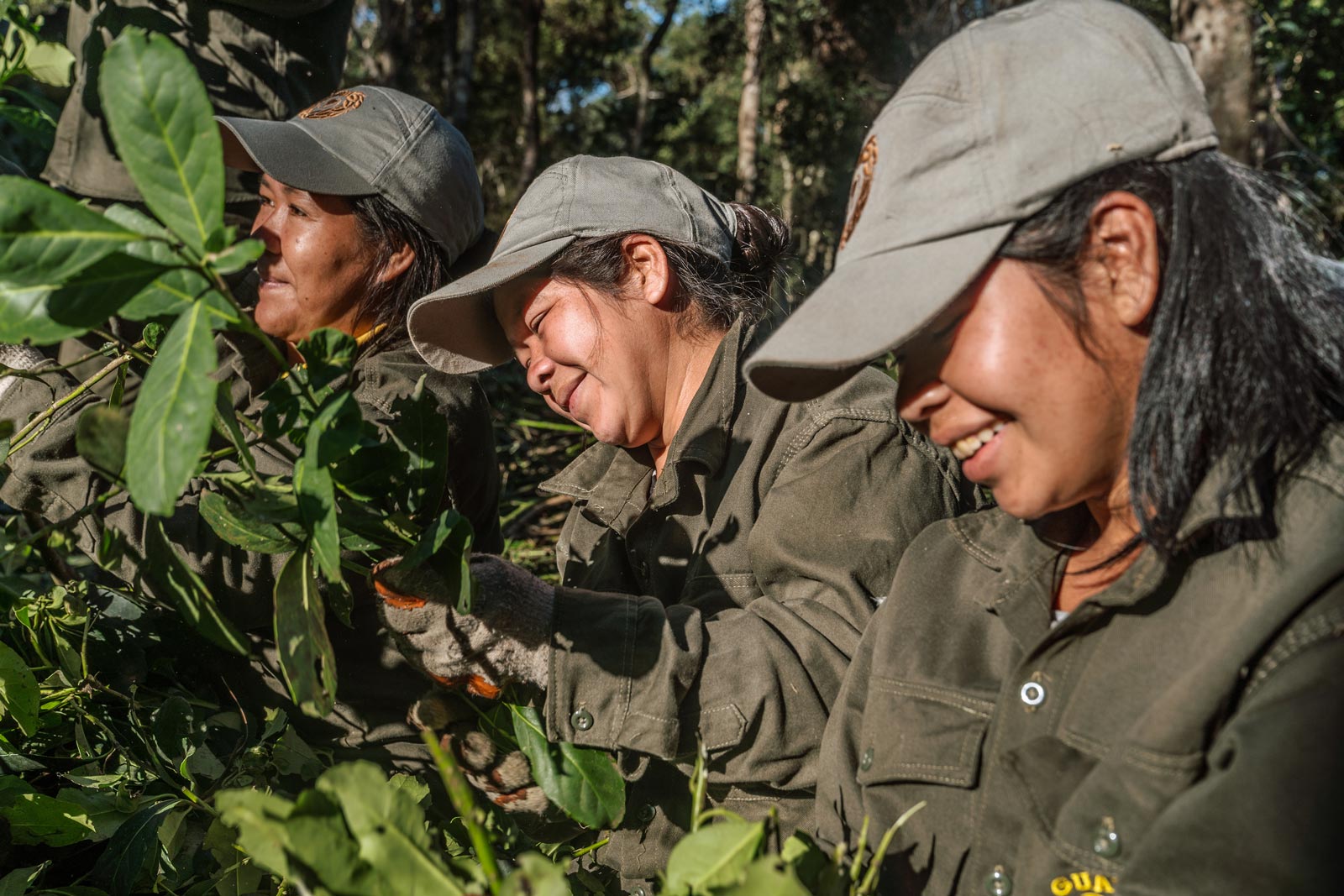This horizontally oriented outdoor photograph captures three women with olive skin and black hair, who appear to be of Spanish descent, engaging in pruning or harvesting activity. They are equipped with gray baseball caps and long-sleeve, dark gray thick cotton shirts that are buttoned up with collars, resembling uniforms. Each woman, visible from the chest up, is either smiling or appearing content as they focus on their tasks amidst large green glossy leaves with oval shapes on green stems. The sun shines from the left side of the image, highlighting the women's diligent expressions and gloved hands tending to the plants. Behind them, a background of trees with thick and thin trunks creates a lush, forested setting. The overall scene depicts a moment of joyful camaraderie and hard work among three happy harvesters.